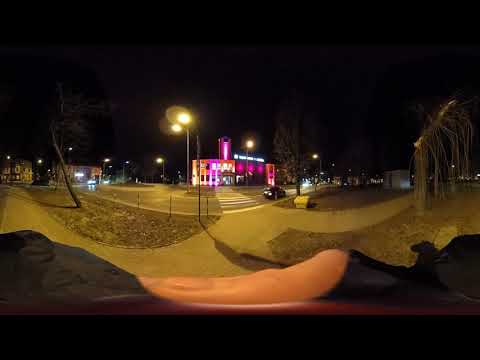The image captures a nighttime city scene with a fish-eye lens effect that curves the scene towards the edges. The perspective is from someone standing on a sidewalk, which has a yellow-amber glow from the surrounding streetlights. A crosswalk marked with white lines leads to a street that stretches out in front, lined with yellow-lit streetlights. To the sides of the road, patches of grass and trees can be seen. Prominently featured on the corner across the street is a building bathed in vibrant purple lighting, which even illuminates a tower at its peak. The image is enveloped in the dark of a completely black sky, accentuating the warm streetlights and the building’s striking purple glow.